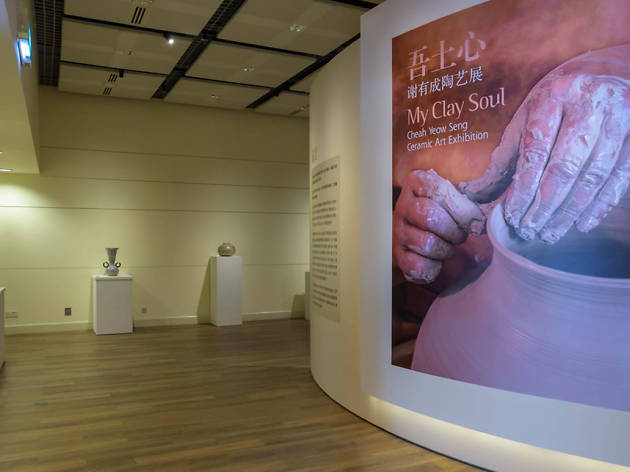The image depicts a museum exhibition titled "My Clay Soul" by Chia You Sung, held in a smaller gallery or museum. The room features a rounded center wall displaying a large, warm-toned banner with Chinese script, alongside an image of two hands crafting a clay pot. The exhibition space is sparse, with ceramic sculptures placed individually on small pedestals, each illuminated by track lighting. The walls are a yellow cremation color, and the space is accented by a standard wooden floor with varied shades. An informational poster further elaborates on the exhibited works. The overall setting gives a minimalist yet focused presentation, emphasizing the artist's intricate ceramic creations.